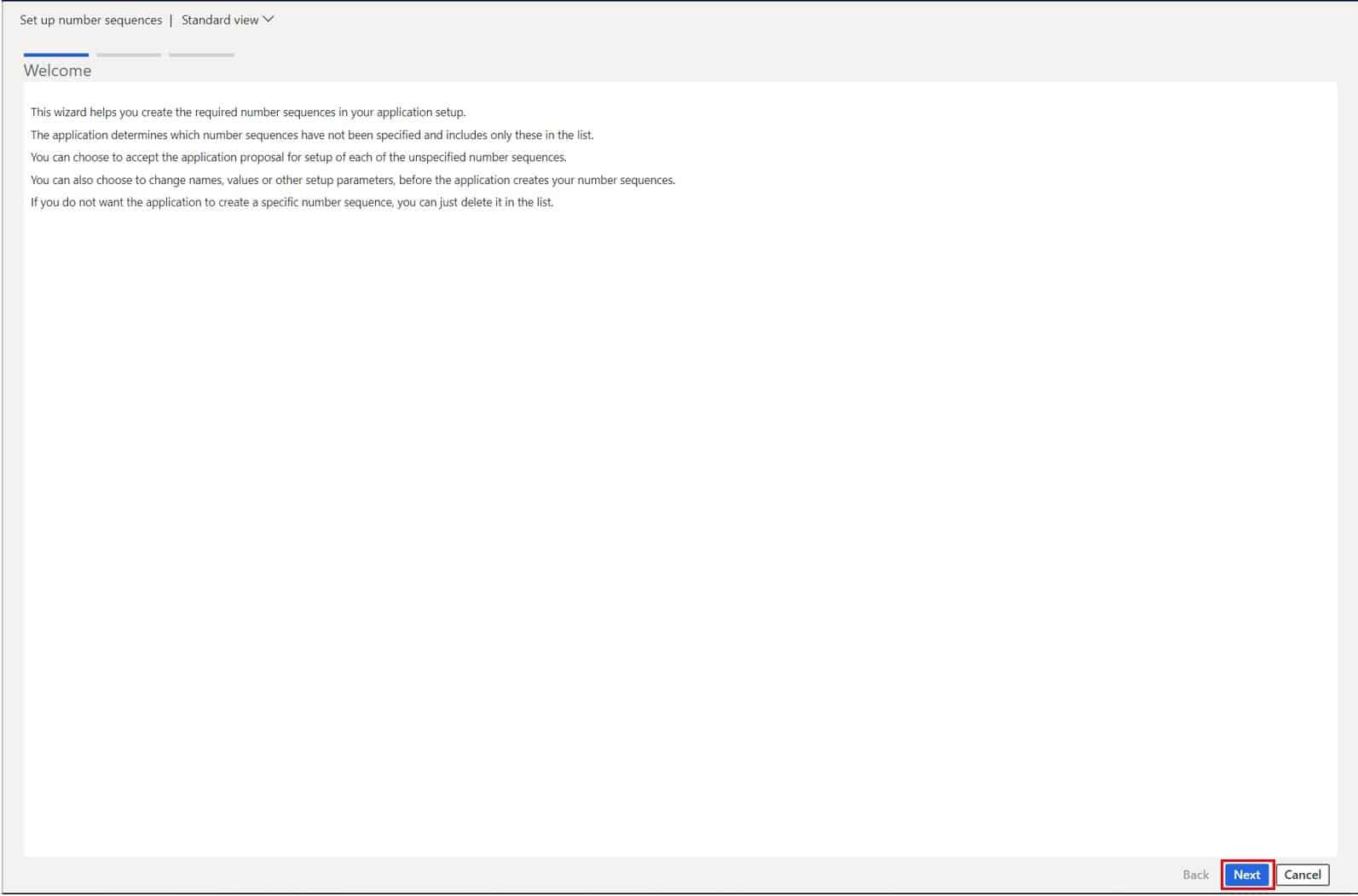A digital image displays an online setup screen for an application setup wizard. The background is completely white, and dark gray text dominates the interface. At the very top, the text reads "Set up Number Sequences," followed by a vertical line and the label "Standard View" accompanied by a drop-down menu arrow. Below this header, there are three horizontal progress indicators side by side; the second and third are grayed out, while the first one is medium blue, indicating the current step.

Beneath the progress indicators is a header labeled "Welcome." Following this are five lines of text that describe the purpose and functionality of this setup wizard. In the lower left-hand corner of the screen, three buttons are visible. The first button, which is grayed out, reads "Back." The second button, prominently highlighted with a red outline, blue center, and white text, reads "Next." The third button, outlined with a thin line and featuring a white background, reads "Cancel."